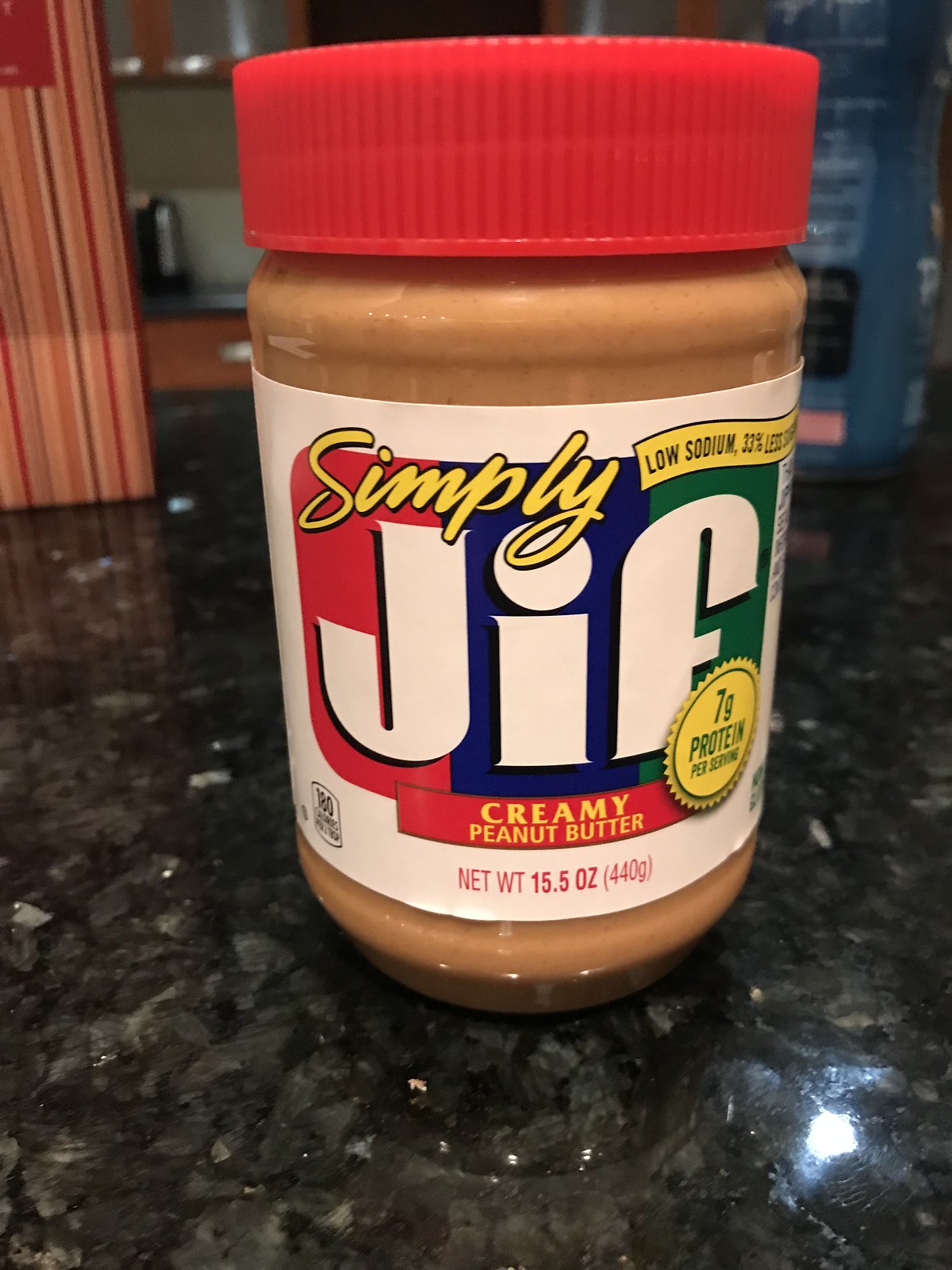A vibrant indoor color photograph captures a neatly arranged jar of peanut butter placed on a sleek, black and gray stone-like countertop. The jar, completely filled to the brim with creamy, light brown peanut butter, stands out prominently against its shiny surface. It is topped with a distinctive red plastic cap, characterized by thin, closely spaced vertical etched lines. The label, wrapping around the jar, features a white background displaying the brand name "Simply Jif Creamy Peanut Butter" and specifies a size of 15.5 ounces. The meticulous details of the presentation enhance the visual appeal, making the jar of peanut butter the focal point against the sophisticated countertop setting.